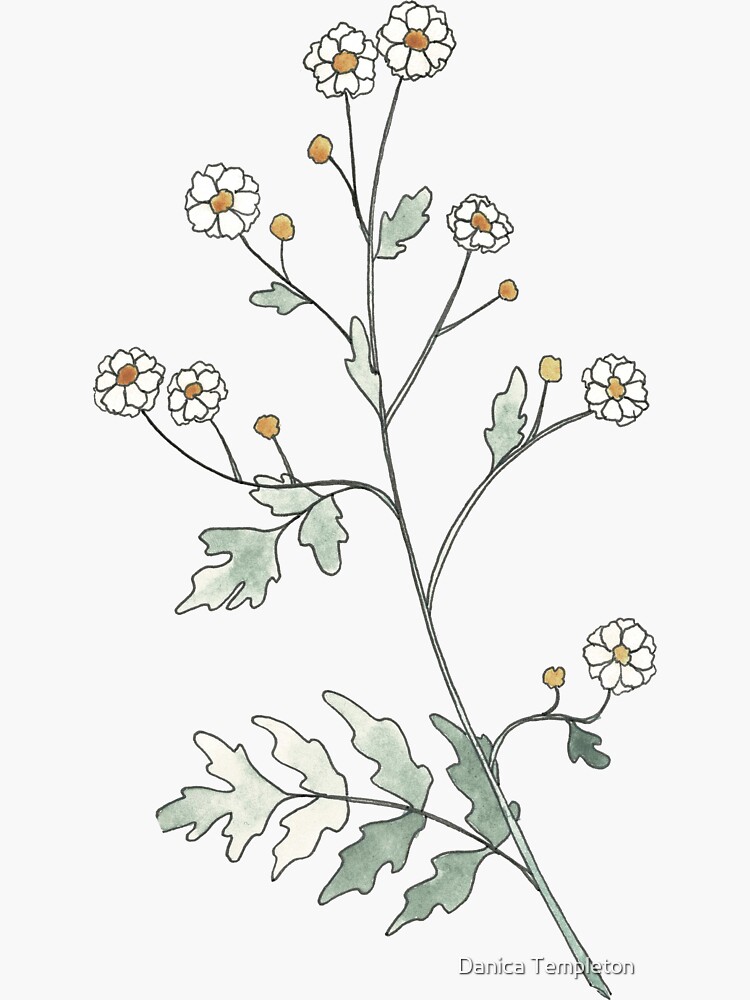This is a digital screenshot of a hand-sketched watercolor artwork by Danika Templeton. The image prominently features a single green stem running from the center of the lower part of the image to the top, adorned with eight fully bloomed white flowers. Each flower showcases short, broad petals with firm, vibrant white coloration surrounding a yellow to orange center. The stem also displays several buds that are in the early stages of blooming, adding a touch of budding potential to the scene. Accompanying the blossoms, the plant is decorated with green leaves that are both fresh and vibrant, resembling fern-like foliage. The artist captures a range of colors including dark green, light green, white, yellow, and gray, portraying the flowers, branches, and leaves with detailed intricacy.